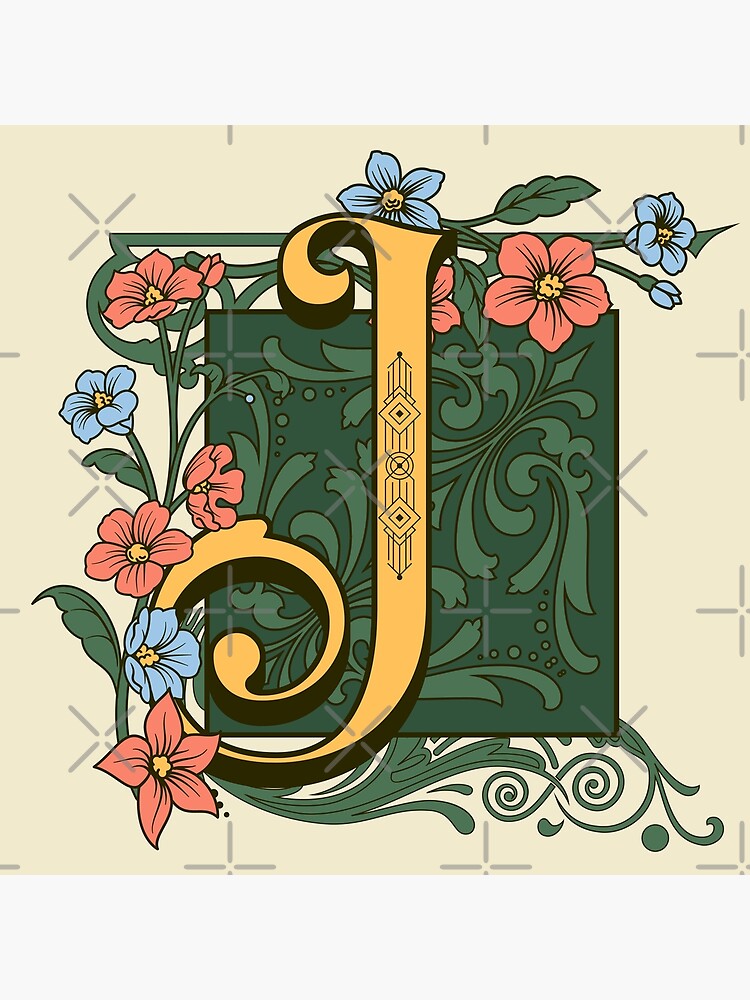The image depicts a detailed, multi-color digital artwork centered around a decorative letter J. The piece is vertically rectangular, with a thick gray border at the top and a light pinkish background. The main focal point is a golden, ornate letter J, set against a green square adorned with a floral design. This golden J features intricate etching, including vertical lines, diamonds, circles, and geometric patterns like triangles and squares, creating a textured appearance. The letter itself displays sophisticated medieval-style script with curved flourishes at both the top and bottom.

Surrounding the letter J is a border of vibrant flowers, which include red, pink, blue, yellow, and tiny purple flowers with green leaves and stalks, creating a rich and colorful frame. The green square the J sits upon resembles a banner with leaf designs varying in size, adding to the intricate nature of the artwork. Additionally, an alternating pattern of watermarked plus signs and X's is scattered across the image, serving as a protective measure to prevent unauthorized duplication.